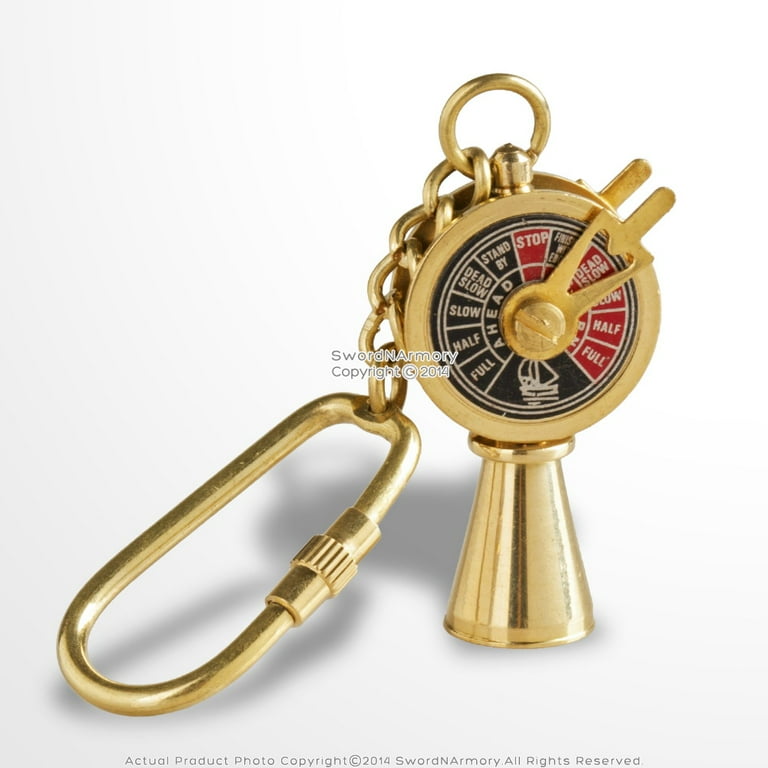The image showcases a shiny and detailed nautical-themed keychain that appears quite hefty. The keychain is gold-colored with a brass-toned large carabiner on the left, connected by chain links to a maritime dial. This dial is split into two halves with a black and red face. The outer rim of the dial features various speed indicators including: "dead slow," "stand by," "stop," "half," "full," and "ahead," in white lettering. At the six o'clock position of the dial, there is a black segment with an image of a sailboat. Surrounding the keychain, there is a small dark gray text at the bottom of the image which reads, "Actual product photo copyright 2014 Sword and Armory all rights reserved."